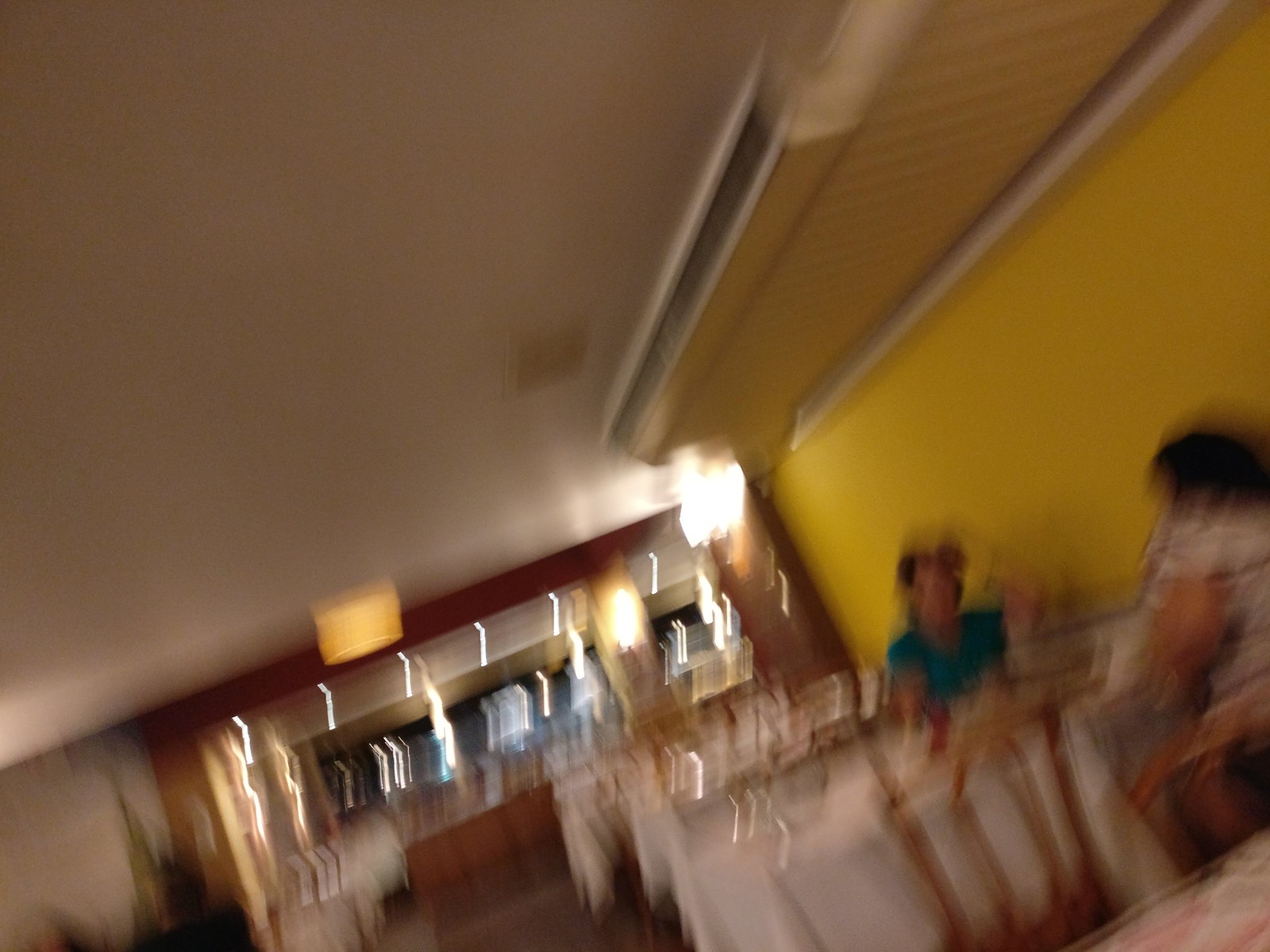A blurred, out-of-focus photo captures the inside of a restaurant from an off-kilter angle, making the space appear as though it’s tilting to the left. On the right side of the image, a white-tableclothed table seats two diners, one in the bottom right corner and one across from them. The table features unoccupied wooden chairs on its left side. The diners’ glasses subtly reflect the ambient light. Behind them, a large yellow wall adds a splash of color to the scene. A prominent light fixture hangs from the ceiling, though this side of the room remains relatively dim. In the center background, another dining area with similarly draped white tablecloths can be vaguely discerned through the blur. The ceiling appears to be lined with white lights that streak due to the camera's unsteady capture.